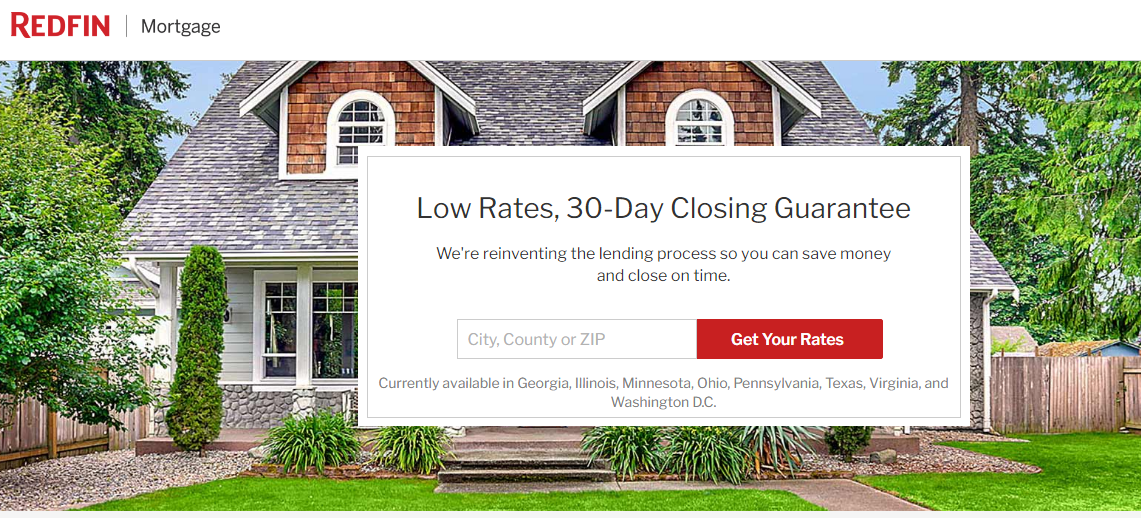This is a detailed screenshot from a website featuring a prominent advertisement for Redfin Mortgage. The top left corner showcases a white background with a red line of text displaying the name "Redfin," adjacent to a vertical gray line separating it from black text that reads "mortgage." Below this header is a photograph of a beautiful home, featuring a bright green lawn extending from the bottom to the bottom right corner. The house itself has a robust stone base, with wood slats above and white-trimmed windows. The roof includes several bump-outs with cedar fronts, also trimmed in white, and is complemented by white gutters. The scene is framed by lush, vibrant green trees on both the left and right sides.

Centrally positioned over the photograph is a prominent white rectangular pop-up ad with a delicate inset light gray border. At the top of the pop-up, large black text boldly proclaims "Low Rates, 30 Day Closing Guarantee." Below this, smaller text states, "We're reinventing the lending process so you can save money and close on time." Further down, there's a light gray text box prompting with "City, county, or ZIP," situated next to a striking red button that features white text saying "Get your rates." 

The bottom section of the pop-up contains small light gray text across two lines, indicating the service is "Currently available in Georgia, Illinois, Minnesota, Ohio, Pennsylvania, Texas, Virginia, and Washington DC." This pop-up takes up a significant portion of the image, obscuring the house from the left window to the right side, while still allowing a glimpse of brown concrete steps beneath it.